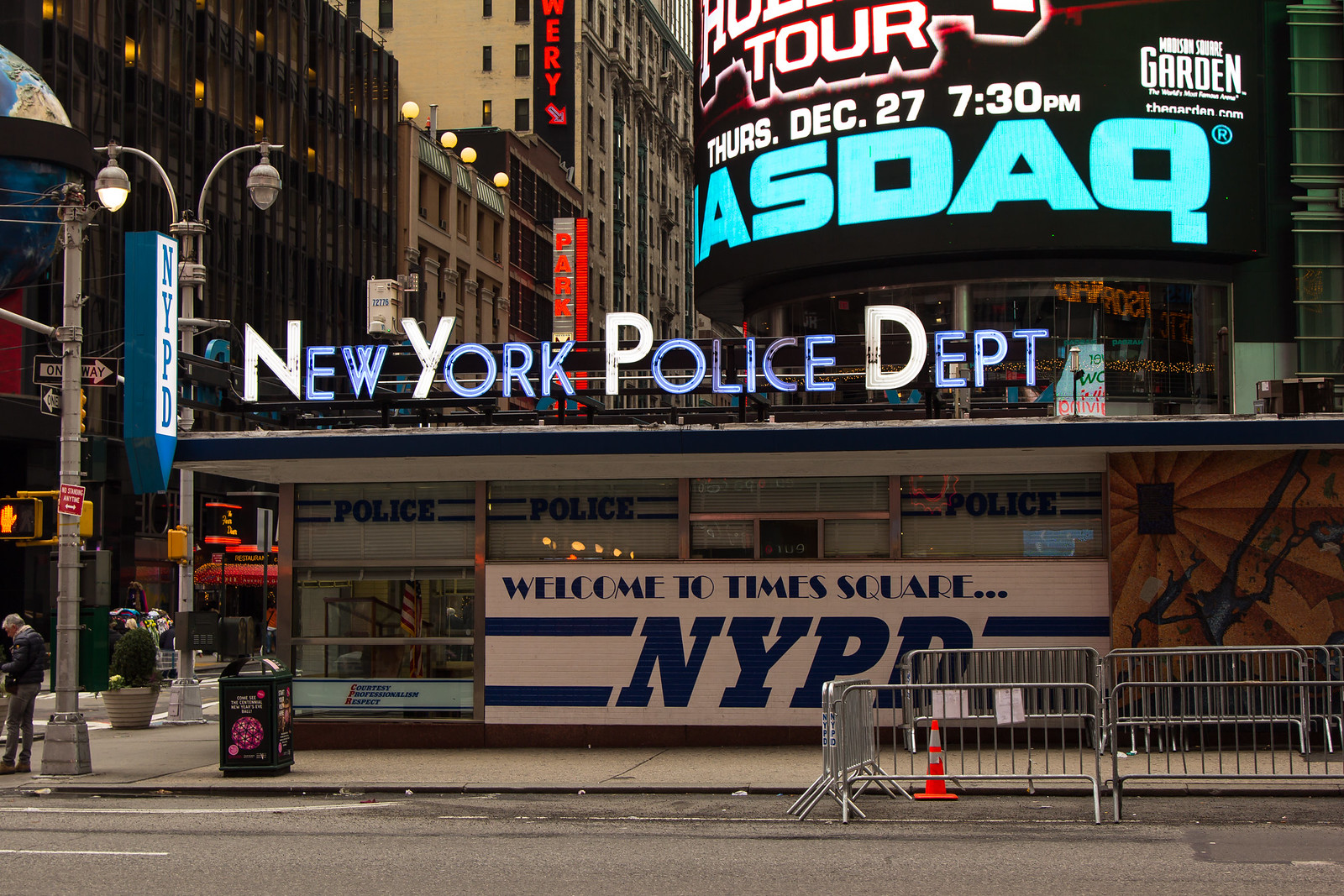This outdoor image captures a bustling street scene at Times Square with a prominent focus on the New York Police Department building. The rectangular building features a simple flat roofline, with "New York Police Department" prominently displayed at the top— the initials "NYPD" in white and the rest of the letters in blue. Below this, a tiled area bears the message "Welcome to Times Square, NYPD" in blue, and the frontage is glass, partially covered by blinds.

In the foreground, there's a street with visible elements such as a street sign, light posts, fencing, cones, and a newspaper stand. A person can be seen waiting to cross the street. The left corner of the image shows a few people near the street corner.

In the background, numerous tall buildings frame the scene; while not all are skyscrapers, one central building towers beyond the image’s edge. Among the signs, a large one on the upper right reads "Tour Thursday, December 27th, 7:30 p.m. Madison Square Garden" with "NASDAQ" in big blue letters below. The scene is further detailed with black lights and an NYPD light in blue, emphasizing the busy urban environment.